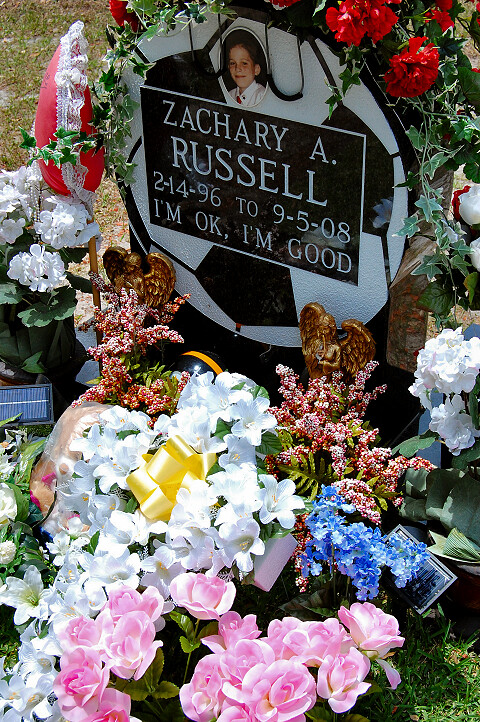The image depicts a somber yet vibrant gravesite for a young child, Zachary A. Russell, who lived from February 14, 1996, to May 29, 2008. The headstone is uniquely shaped like a black and white soccer ball, a possible homage to a beloved sport. At the top of the gravestone is a framed portrait of Zachary. Below the portrait, etched in a black rectangular plaque with white text, are his name, "Zachary A. Russell," and the dates of his birth and passing. Below these details, the reassuring words, "I'm okay, I'm good," are inscribed. Surrounding the gravestone is a profusion of flowers, including red and pink roses, blue blossoms possibly resembling bluebells, and other white and pink flowers intermingled with green foliage and ivy. Two gold angel statues stand vigil at the base of the headstone, flanking either side. To the left, a heart-shaped pillow with lace accents adds a personal touch. The grave is set in a grassy section of a cemetery, with green grass visible in the background and corners of the image.